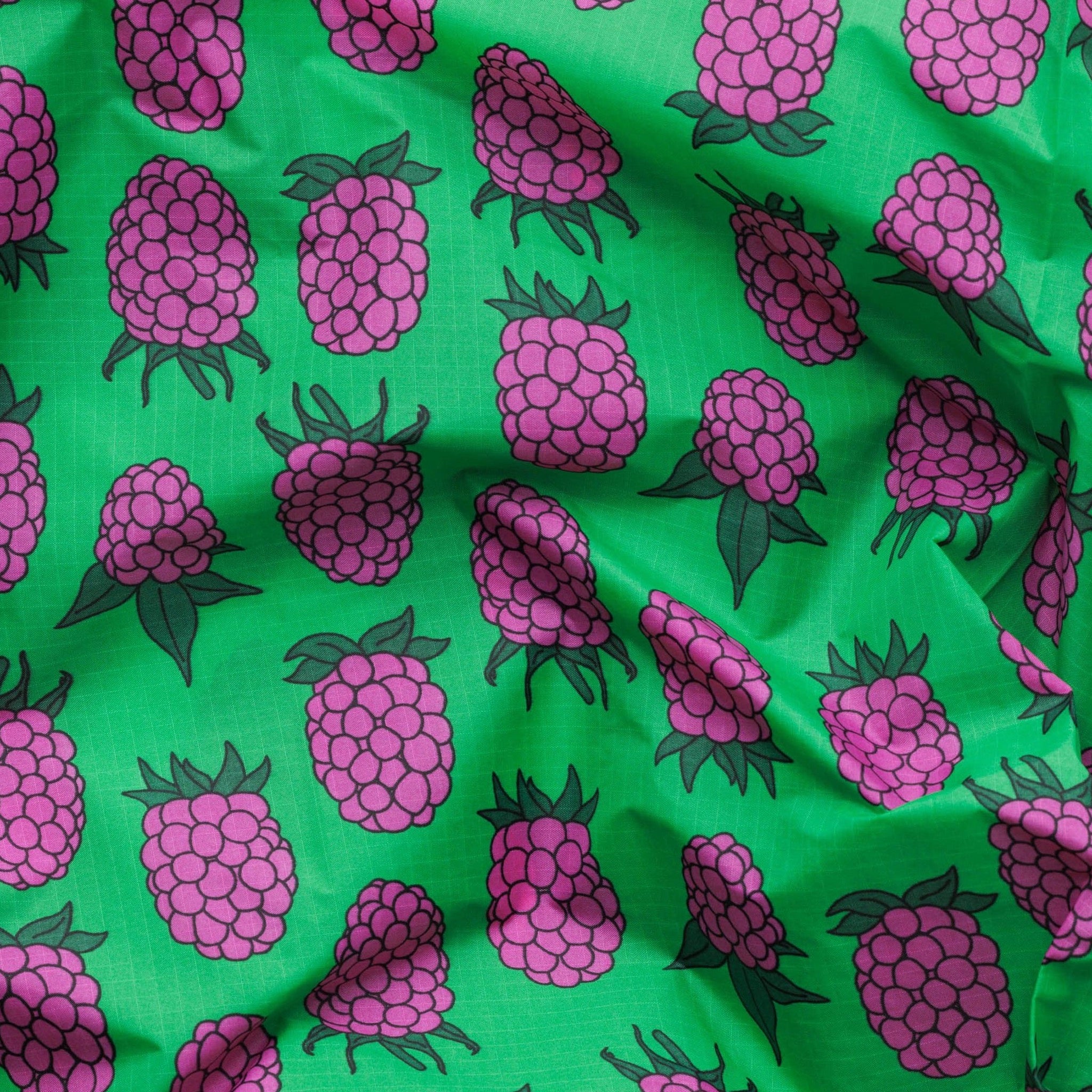This square image, resembling a realistic photograph, features a piece of green fabric, specifically a kelly green hue reminiscent of St. Patrick's Day themes. The fabric is adorned with a lighter green grid pattern, creating a subtle, almost hand-drawn effect. Scattered across the fabric are clusters of purple berries, likely representing either raspberries or grapes, each outlined in black for definition. These berry clusters are detailed with small individual circles and topped with green leaves, varying between four to five leaves per cluster. The image captures the fabric hanging with noticeable folds and creases, particularly crinkled on the right side and slightly wrinkled at the center. The contrasting colors of the purple berries against the green background give it a vibrant and somewhat clashing appearance, making it suitable for use in textiles like sheets or blankets, or potentially in a bold Hawaiian shirt design.